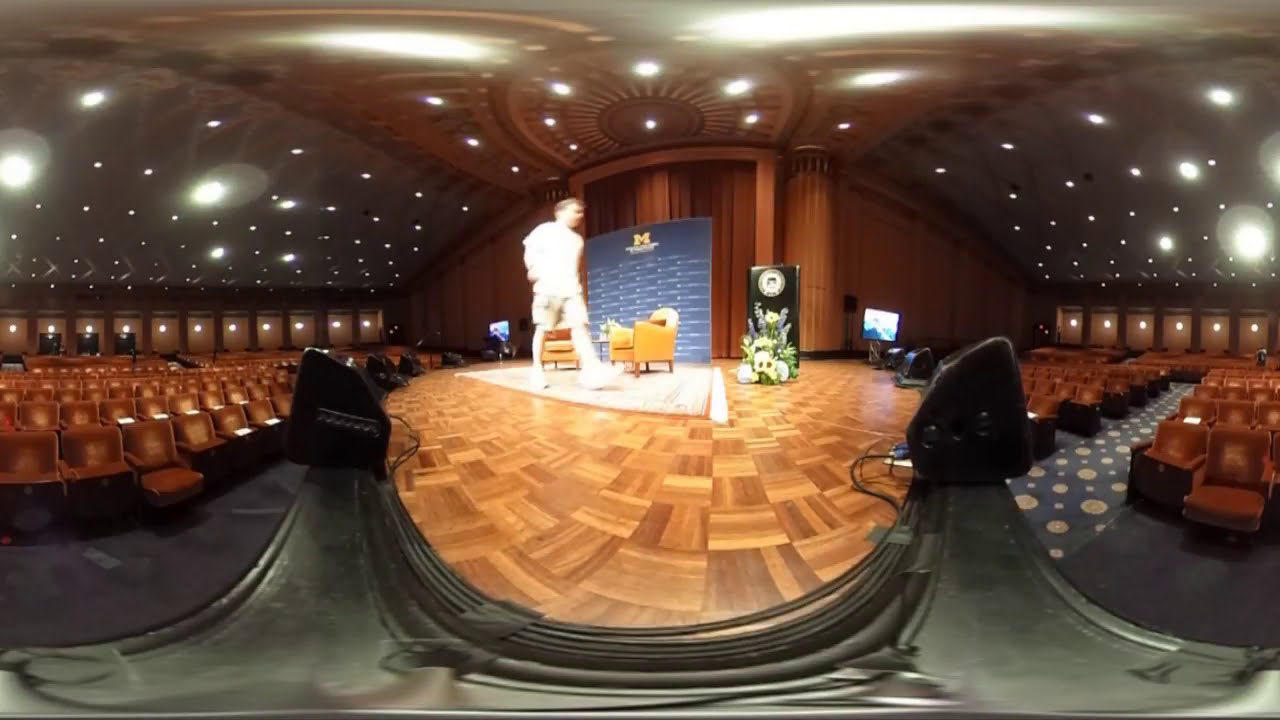In this image of an auditorium, the focus is on a central stage with a parquet wooden floor and a light-colored rug that has two upholstered chairs arranged on it. Atop the rug, a person dressed in a white t-shirt and shorts is walking from left to right, possibly setting up for a presentation. The backdrop of the stage features a large blue board prominently displaying a yellow 'M,' which is likely the University of Michigan emblem, along with other writing that is not legible. The stage is flanked by big black structures that appear to be speakers and additional equipment. To either side of the stage, rows of brown cushioned, stadium-style chairs are situated on an elevated floor covered with dark blue or black carpet. Small spotlights encircle the seating area and stage, their light creating a starry effect on the ceiling. The auditorium's overall layout includes seating that faces inward towards the stage from both the left and right sides, contributing to a focused, intimate atmosphere.